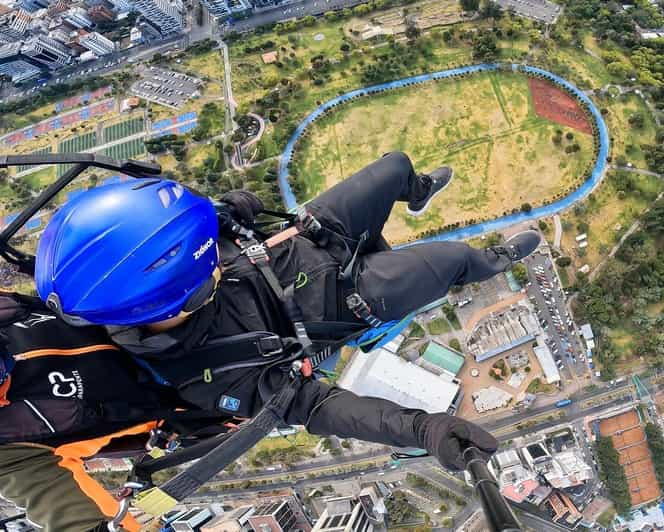In this thrilling photograph, a tandem parachute team is captured mid-descent, with the image taken from a camera mounted on a selfie stick. The primary subject, positioned in a seated posture, is wearing a black jumpsuit and a blue helmet, clearly embracing the exhilaration of the skydive. Behind them, another individual is securely attached, clad in a black suit whose helmet status is not visible. The ground below reveals an intriguing target: an oval-shaped track, possibly a racetrack, inviting speculation about their precise landing zone. The perspective offered by the selfie stick provides a dramatic, bird's-eye view, juxtaposing the skydivers against the sprawling landscape beneath them.